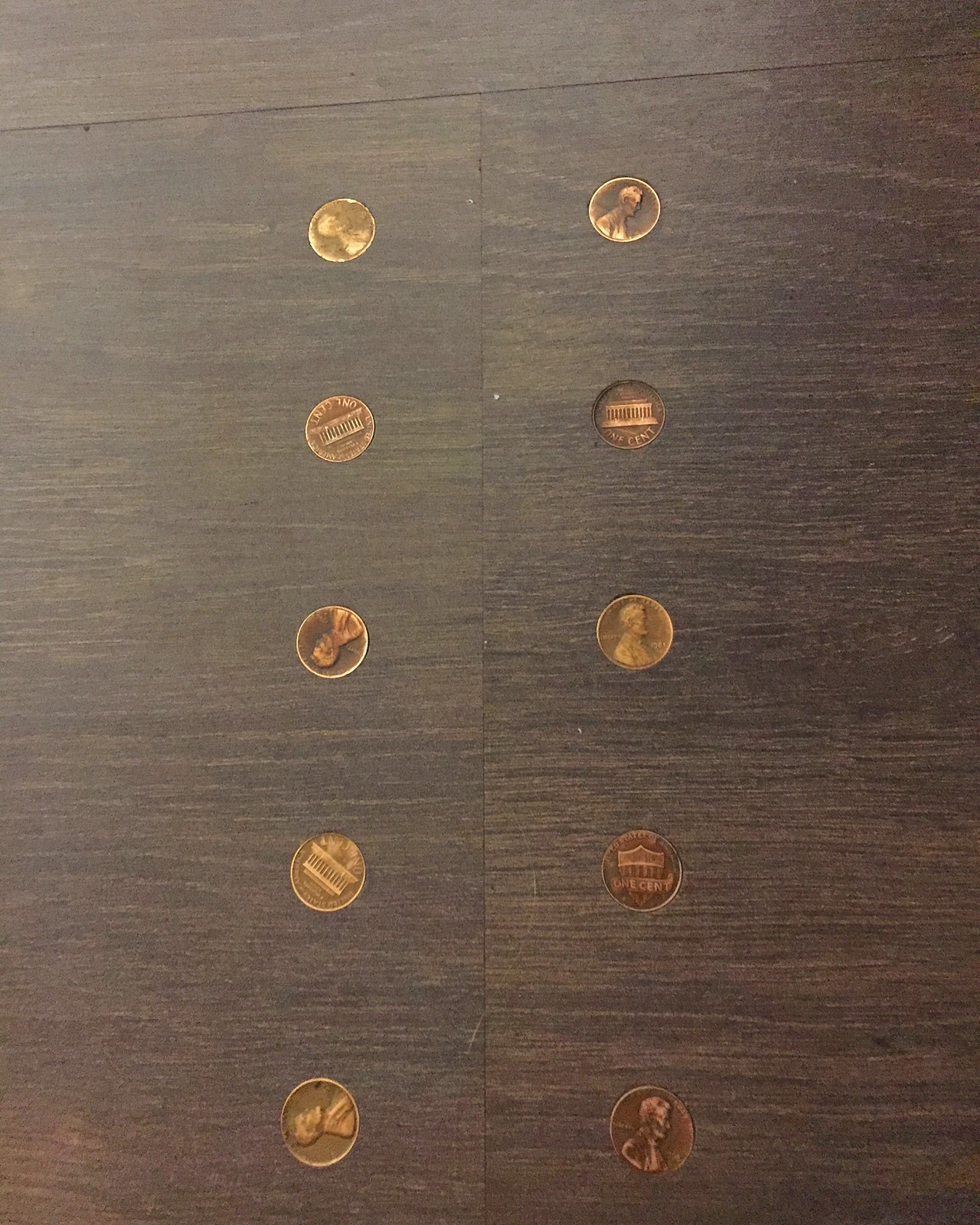On a dark brown laminate table, ten pennies are arranged in a neat grid. The table's surface features a visible T-shaped line pattern that intersects through the middle. The pennies are placed in five rows and two columns. The pennies' orientations vary: in the first row, one penny is heads-up oriented to the left, while the other is tails-up. The second row features an upside-down heads and a tails leaning right. The third row has another heads, oriented straight but towards the front, and a tails directly below it. The fourth row comprises a slightly downward-facing heads and an upside-down tails. At the bottom, there's a heads pointing right and another slightly tilted to the right. Each penny's exact orientation differs, showing heads and tails in various directions and positions across the table.